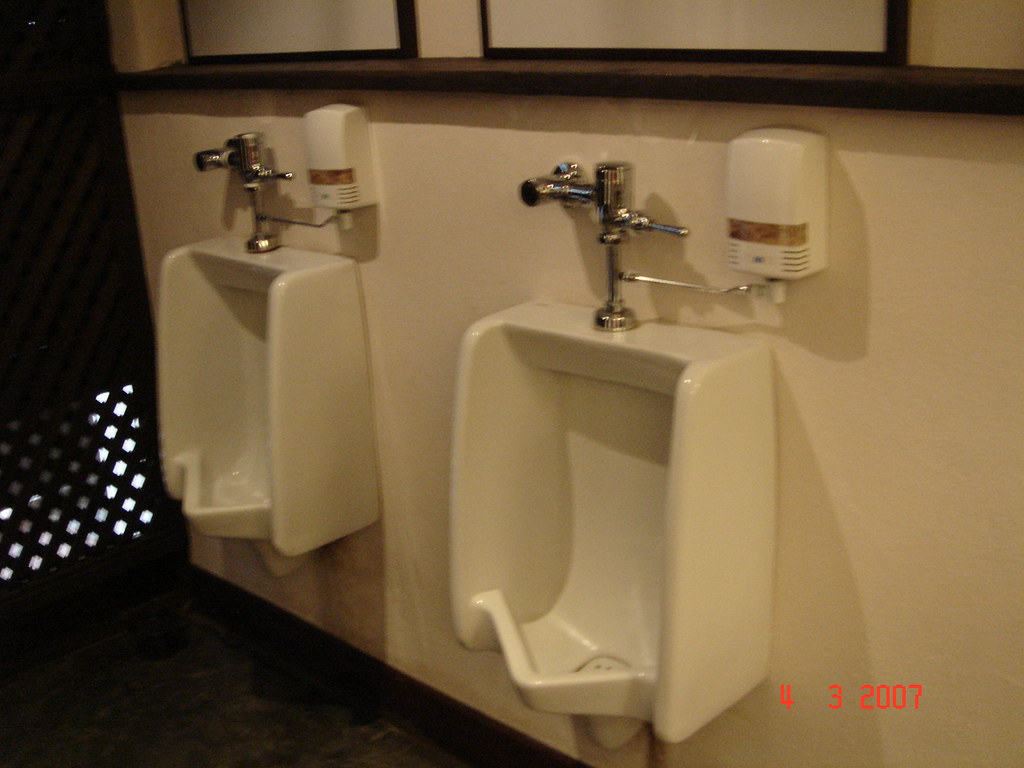The indoor color photograph, captured at a slight angle, features a pair of white porcelain male urinals mounted on a wall that extends larger to the right and recedes towards the background on the left. Each urinal is equipped with a standard chrome flush handle attached to a silver spout protruding from the wall. To the right of the urinals is a shiny white plastic scent dispenser with a yellow see-through band. Above the urinals, there is a dark brown wooden ledge, possibly with mirrors above, although the top part is not clearly visible. The floor in the lower left corner is dark brown, and to the left of the urinals is a brown wall featuring see-through lattice work at the bottom. The image has a slightly grainy texture and a yellowish tint, with an overlay red text date reading "4-3-2007" on the bottom right corner. The background wall is tan, contributing to the overall muted and somewhat out-of-focus appearance of the photograph.